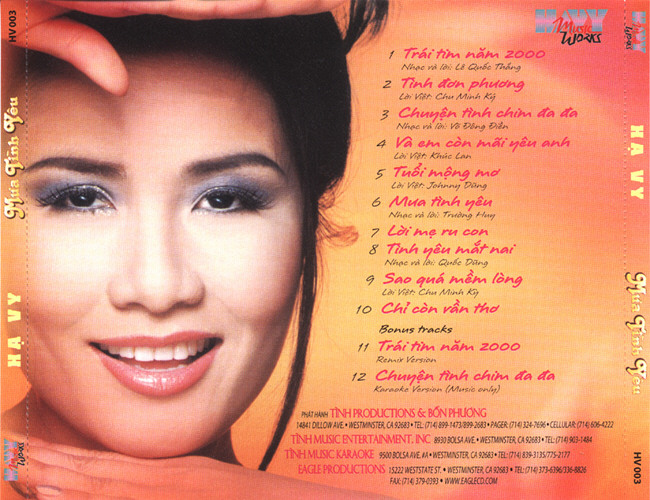The image seems to be an advertisement or the back cover of an LP album, featuring a close-up of an Asian-looking woman with long black hair. She is smiling with her teeth showing and she has bright red lips, emphasized by heavy mascara and eye makeup. Her hair transitions to a bun above her head, and she is posing with her right hand above her face and her left hand extended gracefully under her chin. The background gradient shifts from light to dark peach.

On the right-hand side of the image, there is substantial text content. The upper-right section prominently displays a logo reading "H-A-Y-Y" in large multicolored letters, with the subtext "Music Works" in red and black lettering. Below the logo, there is a numbered list of 12 song titles, all written in an unreadable foreign language. The last two entries are marked as bonus tracks, with additional production information in red and black text at the bottom, detailing the names and addresses of the involved companies.